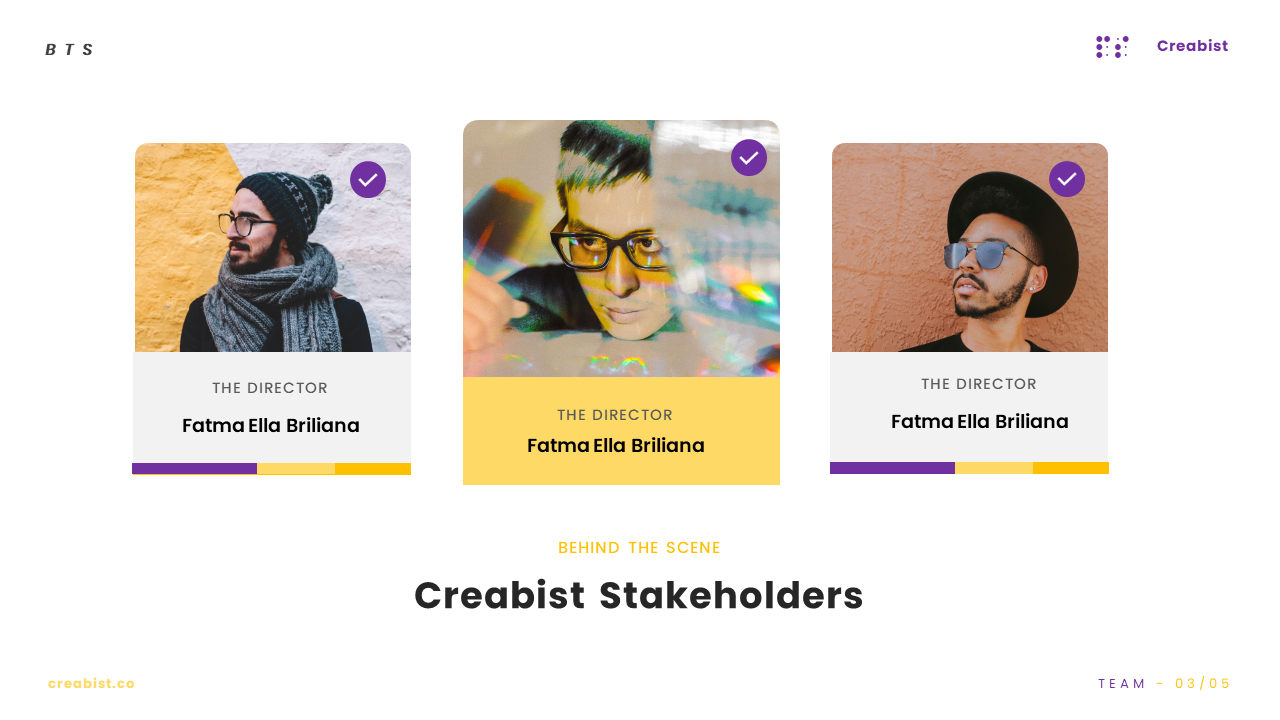The image depicts a webpage layout featuring various sections related to an artistic project or organization. In the top left corner, the acronym 'BTS' is displayed prominently, though its connection to the content is unclear. The top right corner shows the name 'CRABIST' along with the URL 'crabist.co'. In the bottom left section, there is a title that reads 'Behind the Scenes: CRABIST Stakeholders'. Below this title, three individuals are listed with the designation 'Director', each named 'Fatma Ella Bilyana'. This repetition suggests that the names are placeholders, indicating that the actual directors' names have yet to be updated. The overall aesthetic includes a white background, and the image features model-like figures, supporting the theory that this is a preliminary design for a website in development, likely being used to test the functionality and layout of the page.